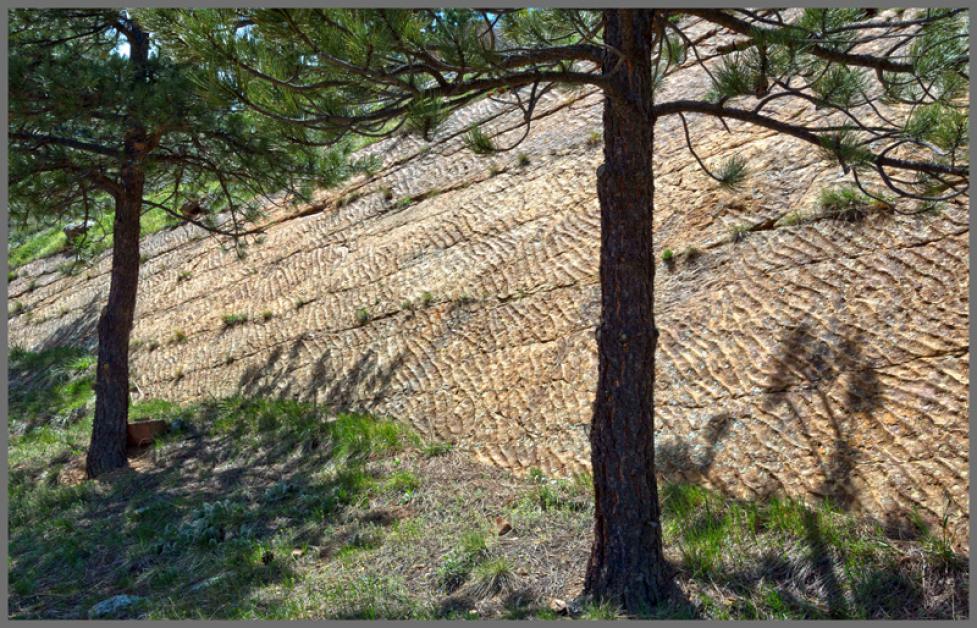This high-contrast photograph, likely taken late in the afternoon given the long shadows, captures the dramatic transition from a forest edge to a sloped, barren hillside. In the foreground, two loblolly pine trees stand tall, their trunks and bottom branches prominently visible with sparse grass and scattered rocks at their base. The hill, slanting to the right and almost desert-like in its pale brown hue, features carved ridges and grooves, with minimal vegetation—only a few sprigs of grass in its cracks. The foreground has slightly more grass but remains patchy, revealing the underlying dirt. Additionally, a small bowl-like object is situated next to the leftmost pine tree, adding a touch of intrigue to the scene.